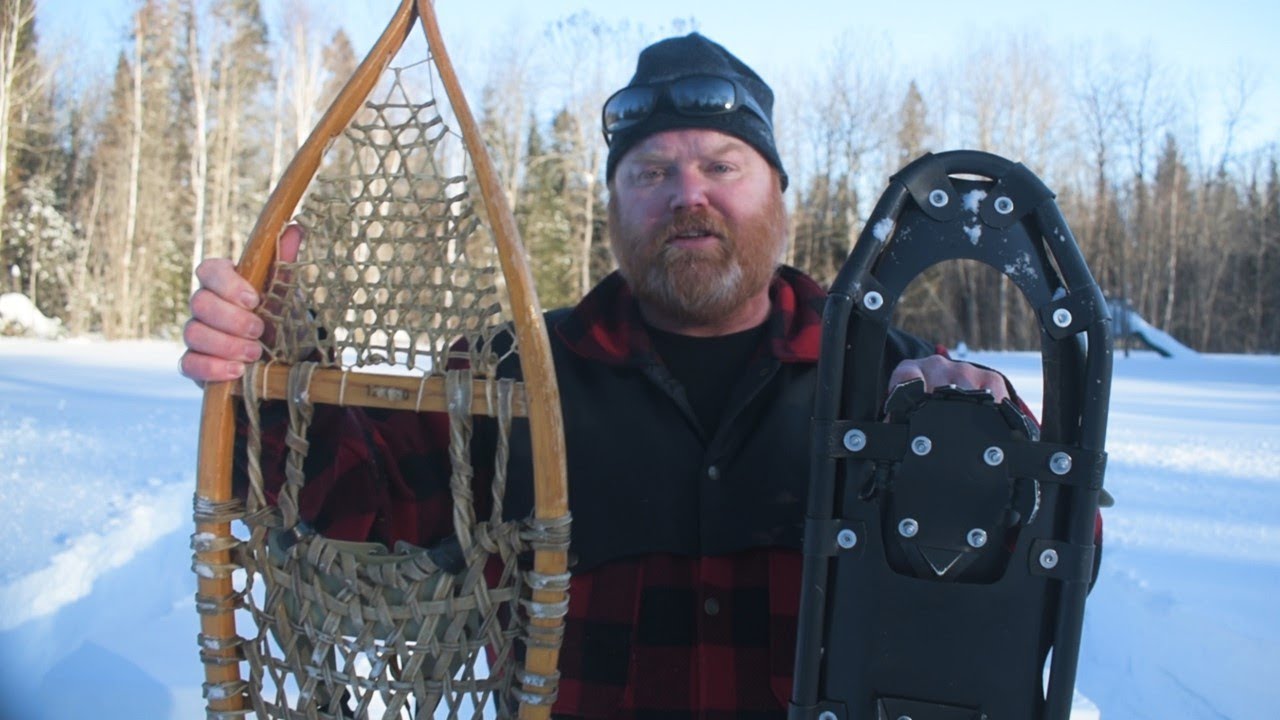A larger white Caucasian man with a red beard, accented with some white on his chin, stands outside in front of a forest on a crisp winter day, the sky a clear blue without a cloud in sight. The ground around him is blanketed in snow. He wears a black ski cap on his head and large sunglasses, perched on the hat. Dressed in a red flannel button-down shirt, his cheeks rosy from the cold, he holds up two different types of snowshoes for comparison. In his right hand, he presents a traditional snowshoe with cloth netting and curved wooden beams forming a leaf-like structure. In his left hand, he displays a modern snowshoe made of black-painted metal, featuring cleats and a lot of screws. The man faces the camera directly, showcasing these contrasting snowshoe styles against the scenic, snowy backdrop.